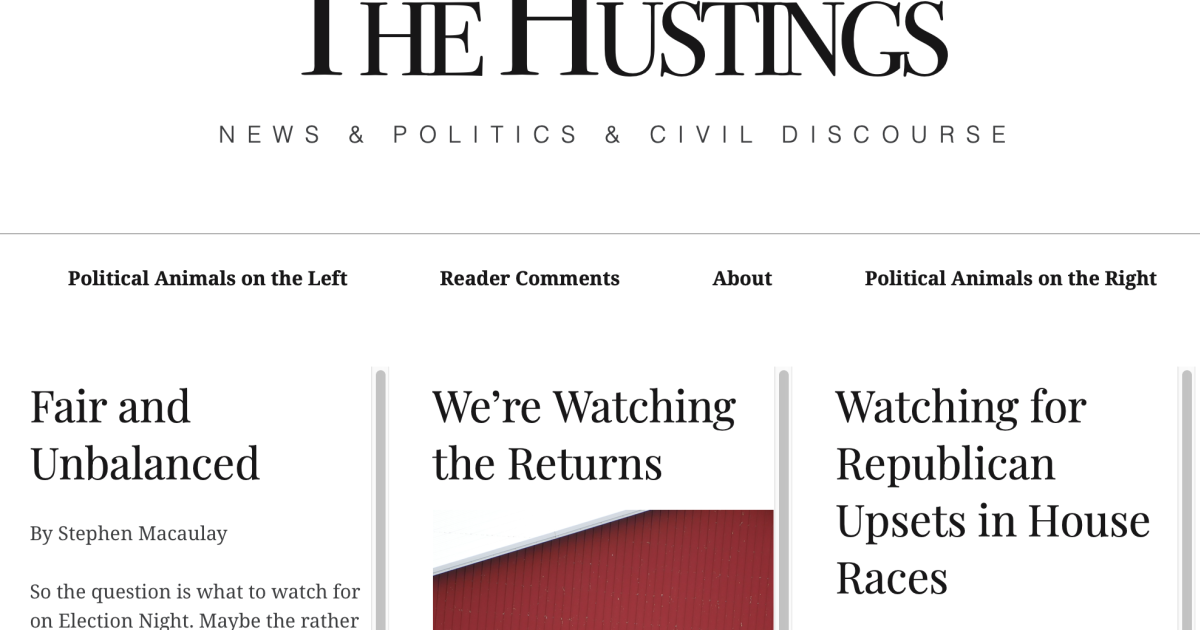This screenshot captures a webpage from "The Hustlings," a site dedicated to news, politics, and civil discourse. The design is minimalist with a clean white background and black text, promoting a professional and readable aesthetic. At the top, the website name, "The Hustlings," is prominently displayed in a large, bold font. Directly beneath it, the tagline "News and Politics and Civil Discourse" succinctly describes the site's focus.

Navigation links are clearly positioned, offering easy access to sections such as "Political Animals," "Reader Comments," and "About." The page's main content area features an array of articles, each presented with a headline, a brief excerpt, and a small image thumbnail. Some of the highlighted articles include "Fair and Unbalanced," "We're Watching the Returns," and "Watching for Republican Upsets in House Races," emphasizing timely and relevant political commentary.

The overall layout is straightforward and user-friendly, allowing visitors to quickly absorb and navigate the content. Even with some portions of the screenshot cut off, it is evident that the site's style is geared towards a professional and news-oriented audience seeking clarity and straightforward presentation.